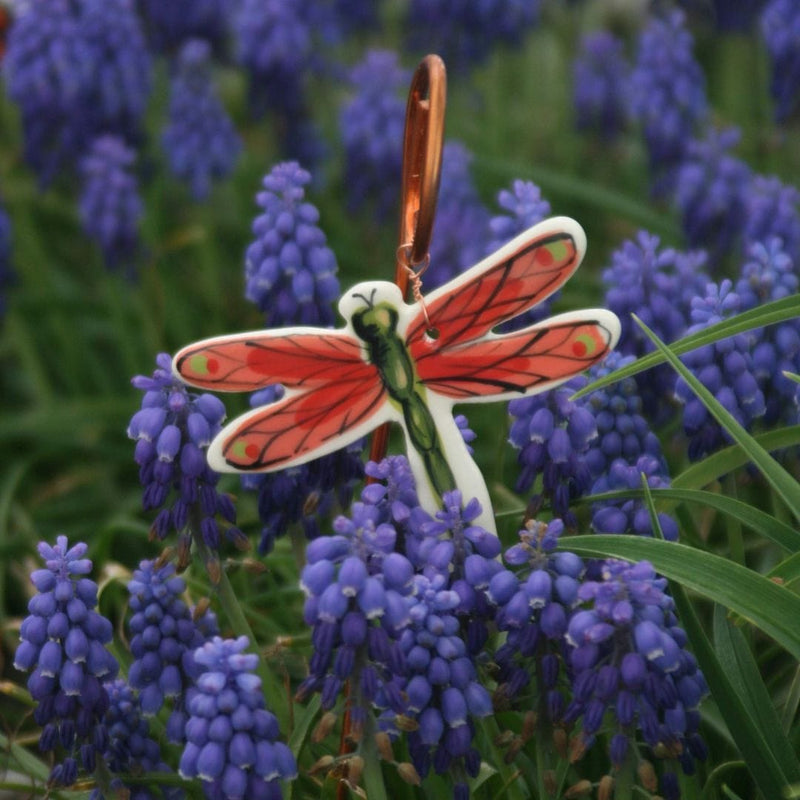In this photograph, there is a detailed scene featuring a lawn ornament amidst a small patch of flowers. The flowers, which are small and abundant, display blue or purple petals and grow on thick green stems, each stem supporting multiple downward-facing blooms. Amongst these blooms, long, dark green grass adds to the lush greenery of the setting. At the center of the image stands a brass rod anchored into the ground, which elegantly curls at the top into a circular design. Suspended from this brass rod by a twisted brass wire is a flat, dragonfly-shaped ornament. This dragonfly is crafted from a white flat piece of plastic and is vividly painted; it has a striking green body and deep red wings. The rustic charm of the brass rod along with the vibrantly painted dragonfly contrasts beautifully with the natural hues of the flowers and grass surrounding it, creating a balanced and serene visual composition.